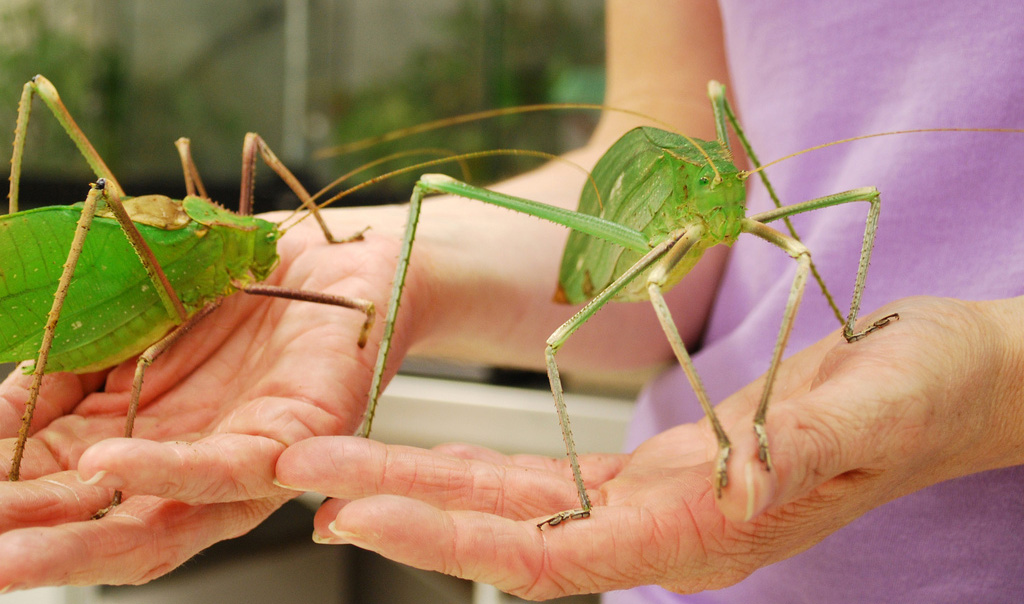In this horizontal rectangular image, we see a woman's hands prominently featured against a blurred background. She is wearing a purple shirt, and her hands are gently cradling two large insects. The insects resemble leaves with their green, leaf-shaped bodies and long, stick-like legs. Each insect has six legs and long antennas, with slight color variations — one being a brighter green and the other a more muted green. The insects' limbs appear brown or tan. The background, though obscured, hints at more green foliage, further emphasizing the natural setting. The focus here is clearly on the woman's hands and the intricate details of these leaf-like bugs she holds.